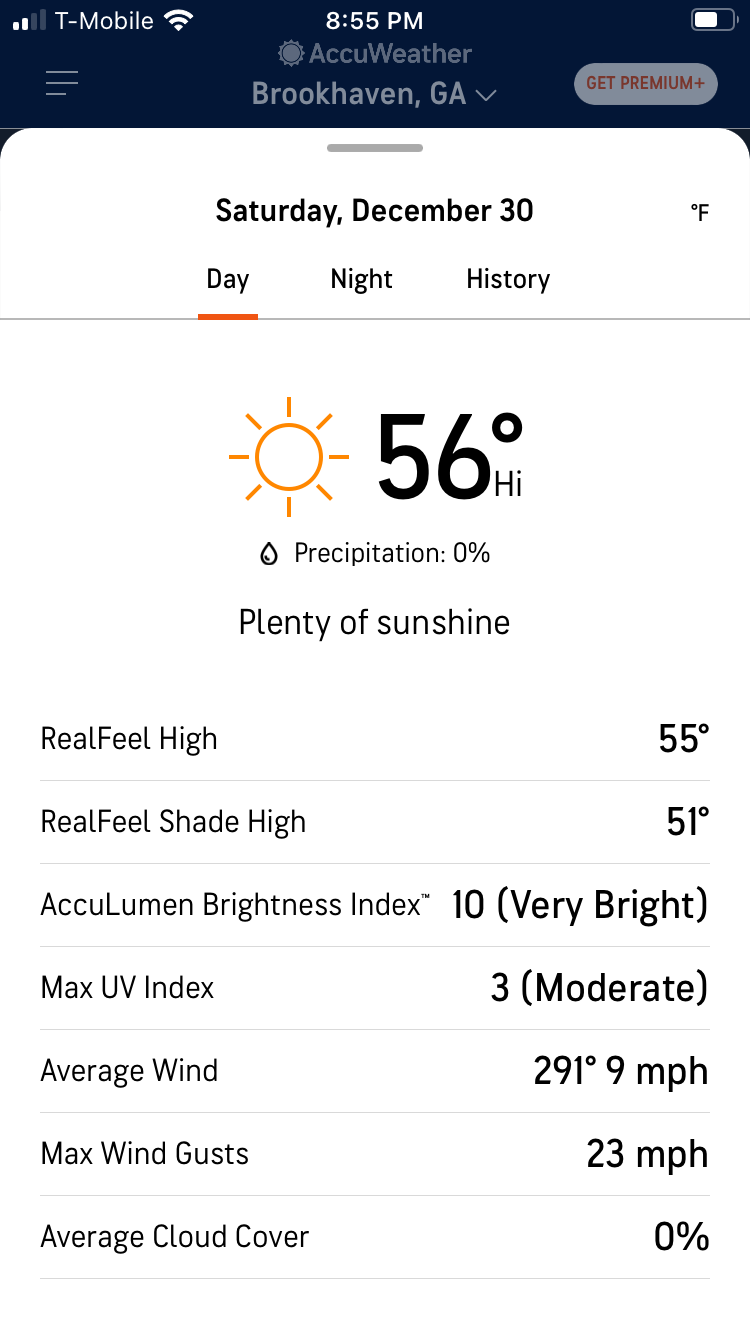The vertical image, captured from a smartphone, predominantly displays a white background likely illuminated by a computer screen. At the top, a dark navy blue rectangle spans horizontally from left to right. On this rectangle, the upper left shows the signal bar strength icon followed by the label "T-Mobile" and the Wi-Fi icon. Centrally positioned in white text, the time reads "8:55 p.m.," while the battery life icon appears on the upper right.

Directly below the navy bar, three horizontal lines, representing more options, are visible. In the middle, the text "AccuWeather" is displayed, indicating the chosen city as "Brookhaven, Georgia," with a "Get Premium" option beside it.

Transitioning to the white background, a thin grey line divides the sections. Below this line, the date "Saturday, December 30th" is displayed in black text. Below the date, the temperature information is provided in degrees Fahrenheit, with "Day" underlined in orange, signifying the selected time period. Other options available include "Night" and "History."

An icon of the sun indicates a high of 56 degrees with 0% precipitation, described as "plenty of sunshine." Further details about the temperature include a "Real Feel" high of 55 degrees, a "Real Feel Shade" high of 51 degrees, and an "AccuLumen Brightness Index" rated at 10, indicating very bright conditions. Additionally, the Max UV Index is listed as three, which is moderate. The wind conditions show an average speed of nine miles per hour at a direction of 291 degrees, with maximum wind gusts reaching 23 miles per hour. Lastly, the average cloud cover is reported to be 0%.